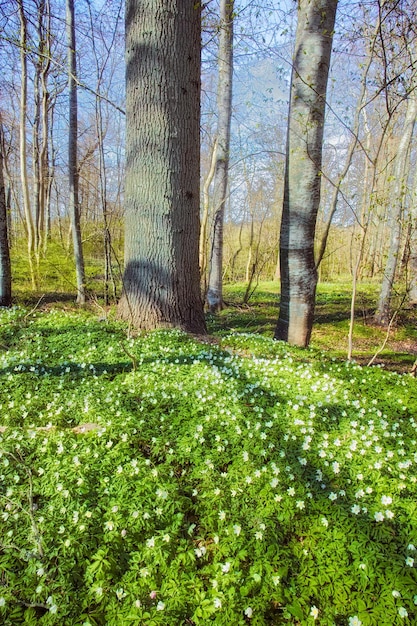The image captures a serene forest glade in what appears to be early spring. In the foreground, dense green moss, intermixed with an abundance of tiny white star-shaped flowers, spreads like a lush carpet. The moss covers about half of the photo, creating a rich, verdant base that contrasts with the bare trunks of surrounding deciduous trees, suggesting they are in a stage before leafing out. Among these trees, an oak stands out towards the left of the center, its robust trunk prominent against a backdrop of thinner, sapling trees that grow densely together. The scene is bathed in soft light, casting subtle shadows on the trunks. Beyond, the mowed yard transitions into an area of overgrown grass, giving way to a mixed array of thin trees. Through the branches, patches of blue sky with light cloud cover are visible, adding to the calm yet vibrant atmosphere of the forest setting.